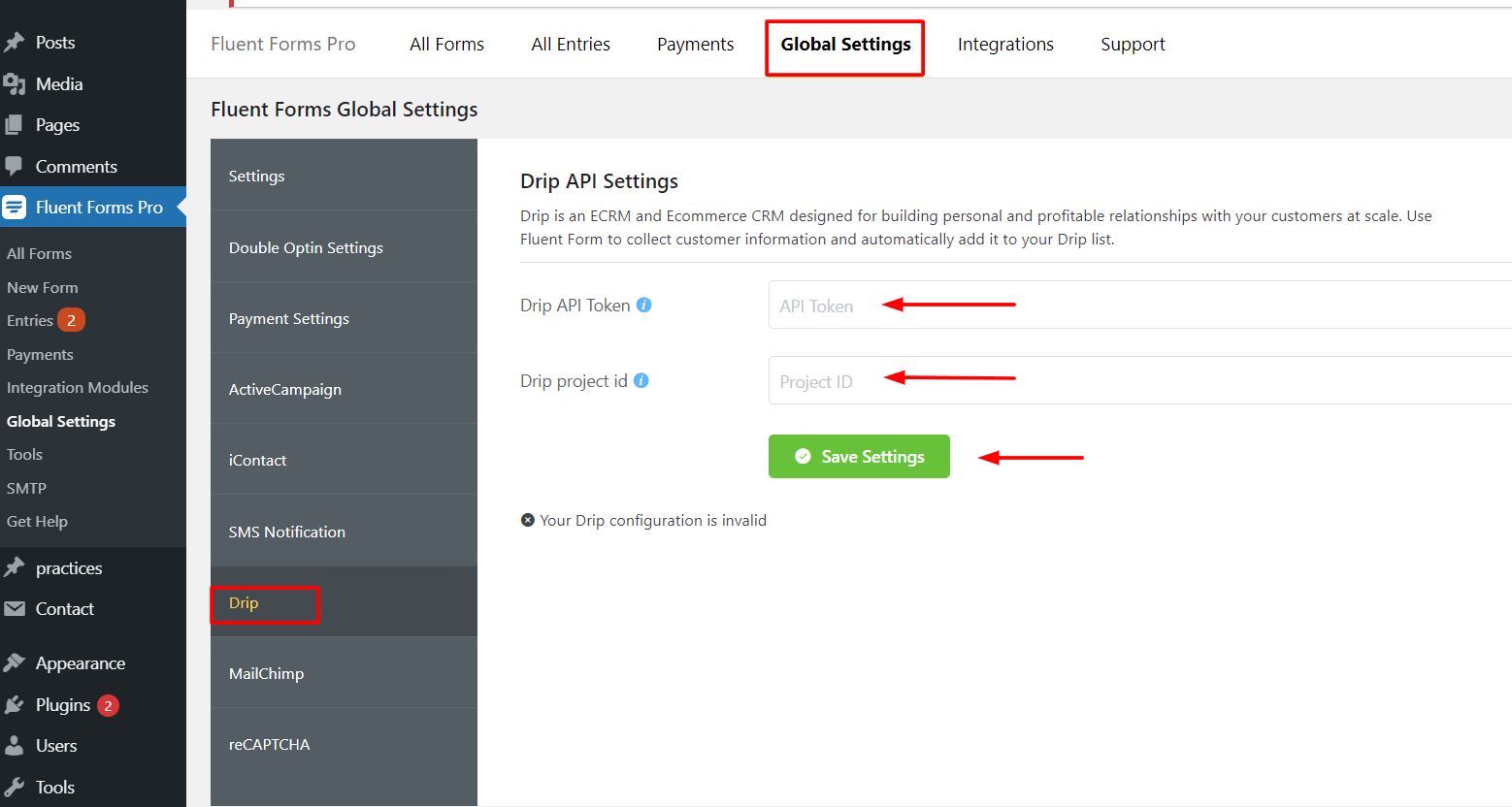On the left side of the image, there is an extensive vertical menu with a dark gray background and white text featuring gray icons. The first menu item, labeled "Posts," is accompanied by a push pin icon, pointing from top right to bottom left. Below that, the "Media" option displays an icon of a camera with a music note behind it. The next item, "Pages," is represented by two overlaid pages. Following is the "Comments" option, depicted with a comment bubble icon.

Further down, a highlighted entry with a white square containing several blue lines reads "Fluent Forms Pro." This option stands out because it is highlighted in blue, featuring an indentation on the right resembling an arrowhead pointing to the left. Activating this option reveals a sub-menu with a medium gray background and white text listing various configurations: "Settings," "Double Opt-in Settings," "Payment Settings," "Active Campaign," "Eye Contact," "SMS Notification," and "Drip." The "Drip" option is distinctly selected, presented with an orange font on a dark gray background, and enclosed by a red rectangular border.

Beneath this, the sub-menu returns to its standard medium gray background with items labeled "MailChimp" and "Recaptcha" in white text. To the right of the menu, the main content area has a white background. At the top left, it reads "Drip API Settings" followed by a smaller gray text explaining, "Drip is an eCRM and eCommerce platform designed for building personal and profitable relationships with your customers at scale. Use Fluent Forms to collect customer information and automatically add it to your Drip list."